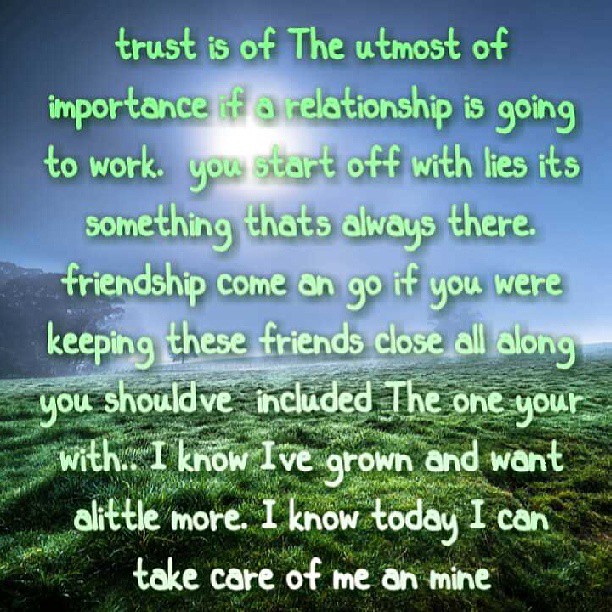The image is an inspirational poster displaying a motivational saying. The text reads: "Trust is of the utmost importance if a relationship is going to work. You start off with lies; it's something that's always there. Friendships come and go. If you were keeping these friends close all along, you should have included the one you're with. I know I've grown and want a little more. I know today I can take care of me and mine." The text is written in green letters that fade from dark at the top to lighter at the bottom.

The background features a lush, green grassy field that looks almost hilly, extending into a backdrop of blue sky. There are a few trees to the left, which have a slightly blue tint. The sun is positioned slightly to the left of the center, creating a bright glare. The overall setting of the poster conveys a serene and optimistic feeling, enhanced by the vivid colors of the bright day.